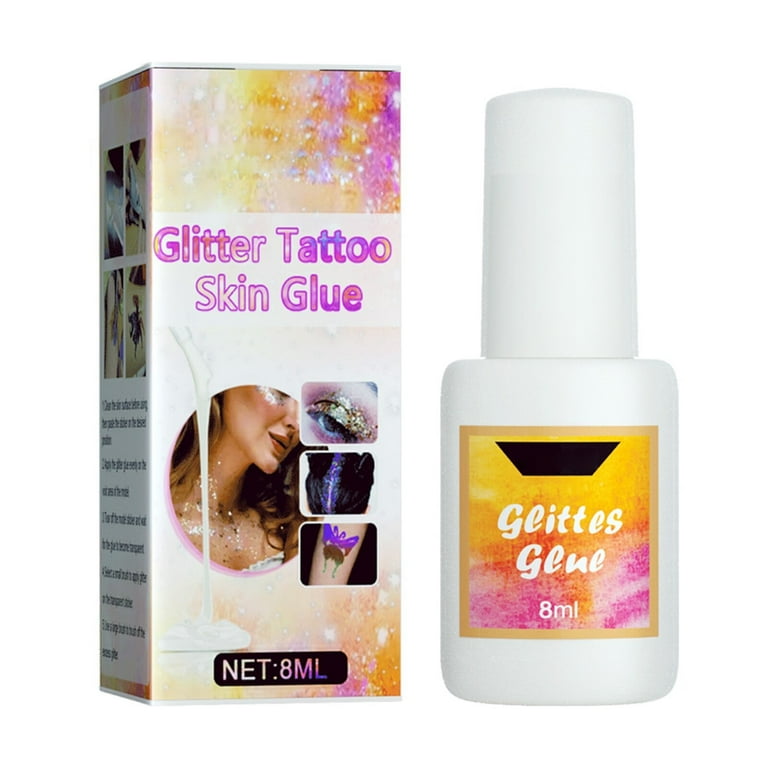In the image, a white bottle and a colorful box are prominently displayed, suggesting a cohesive product package. The bottle features a yellow label with a brown border, adorned with the name "Glittergen" in white lettering, and indicates a volume of 8 milliliters. The box mirrors the bottle’s color scheme with yellow, pink, purple, and gray elements. It prominently reads "Glitter Tattoo Skin Glue" in pink and purple lettering over a white border at the top. 

Below this title, the box showcases various images illustrating the potential uses for the product: decorative glitter applied to areas such as a woman's neck, under her eye, on an eyelid, over her eye, and another unidentified area. The images in the background display a predominantly white palette with splashes of yellow and purple. The glitter appears in various colors, including purple, black, brown, and green, offering versatile application suggestions for the skin glue.